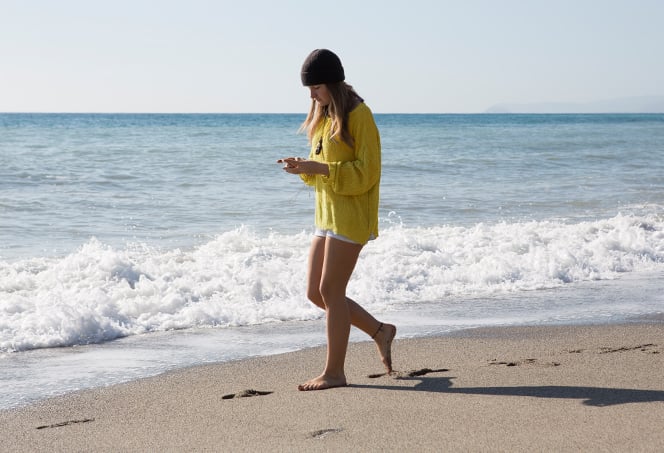The photograph captures a serene daytime scene on the beach, showcasing a young woman walking along the shoreline with a picturesque backdrop of clear blue skies and gentle ocean waves. Centered in the image, the woman is moving towards the left, her right leg poised on its toe and her left foot flat on the sand, leaving behind a trail of footprints. She has shoulder-length brown hair partially covered by a black beanie and is dressed in a long-sleeved yellow sweater paired with white shorts. Her bare feet reveal a delicate anklet, and she wears a prominent necklace. With her hands extended in front of her, she appears engrossed in her phone. The beach's light brown sand stretches up to meet the foamy white surf to her right, with the vast open water extending beyond. The sky above transitions from a light blue to a hazy, almost grayish hue, casting a gentle light that creates a soft shadow on the sand.